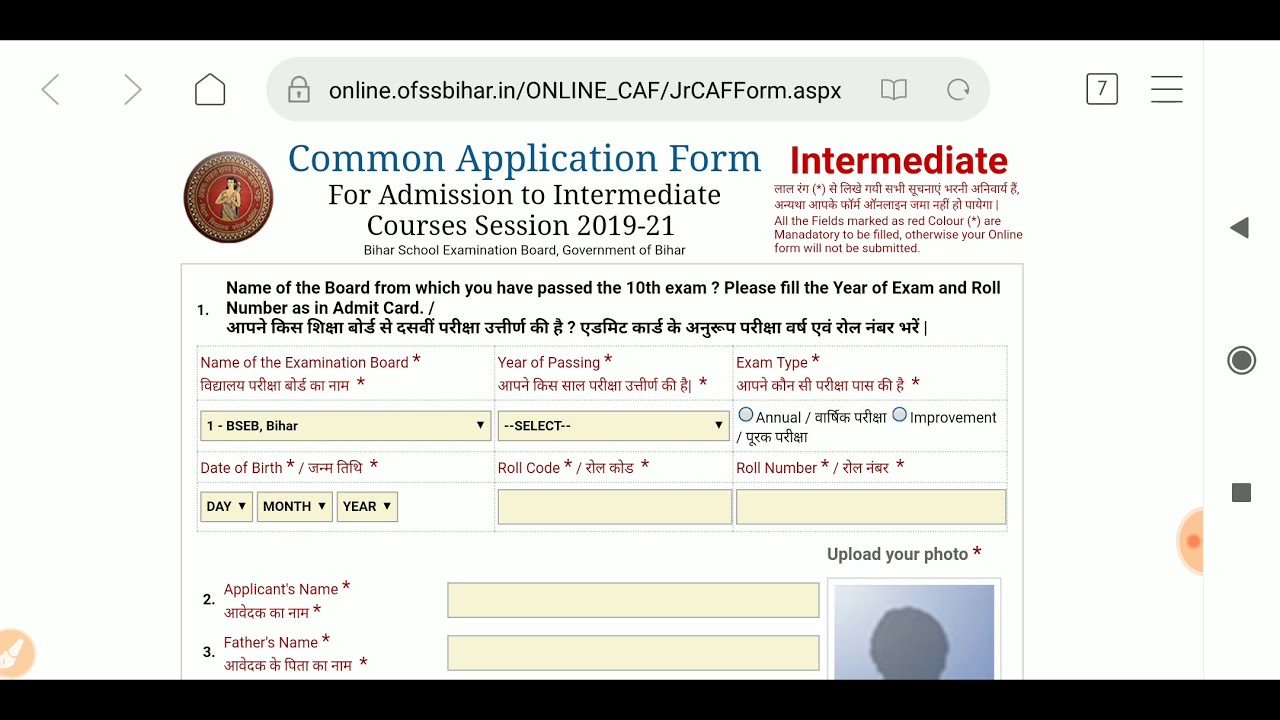The image is a detailed screenshot of a website page displaying the "Common Application Form for Admission to Intermediate Courses, Session 2019-21" from the Bihar School Examination Board, Government of Bihar. The top part of the image features a black bar with navigation icons and a search bar, along with a circular logo on the left. The application form is prominently titled in blue and black text, with "Intermediate" marked in bold red letters in the upper right corner, indicating mandatory fields in red. The form contains several sections to be filled out, including the name of the board from which the 10th exam was passed, year of passing, exam type, date of birth, roll code, roll number, applicant's name, and father's name. There is also a field to upload a photo, currently showing a gray silhouette. The page displays a mix of English text and non-English characters, suggesting it is intended for a non-English speaking region.